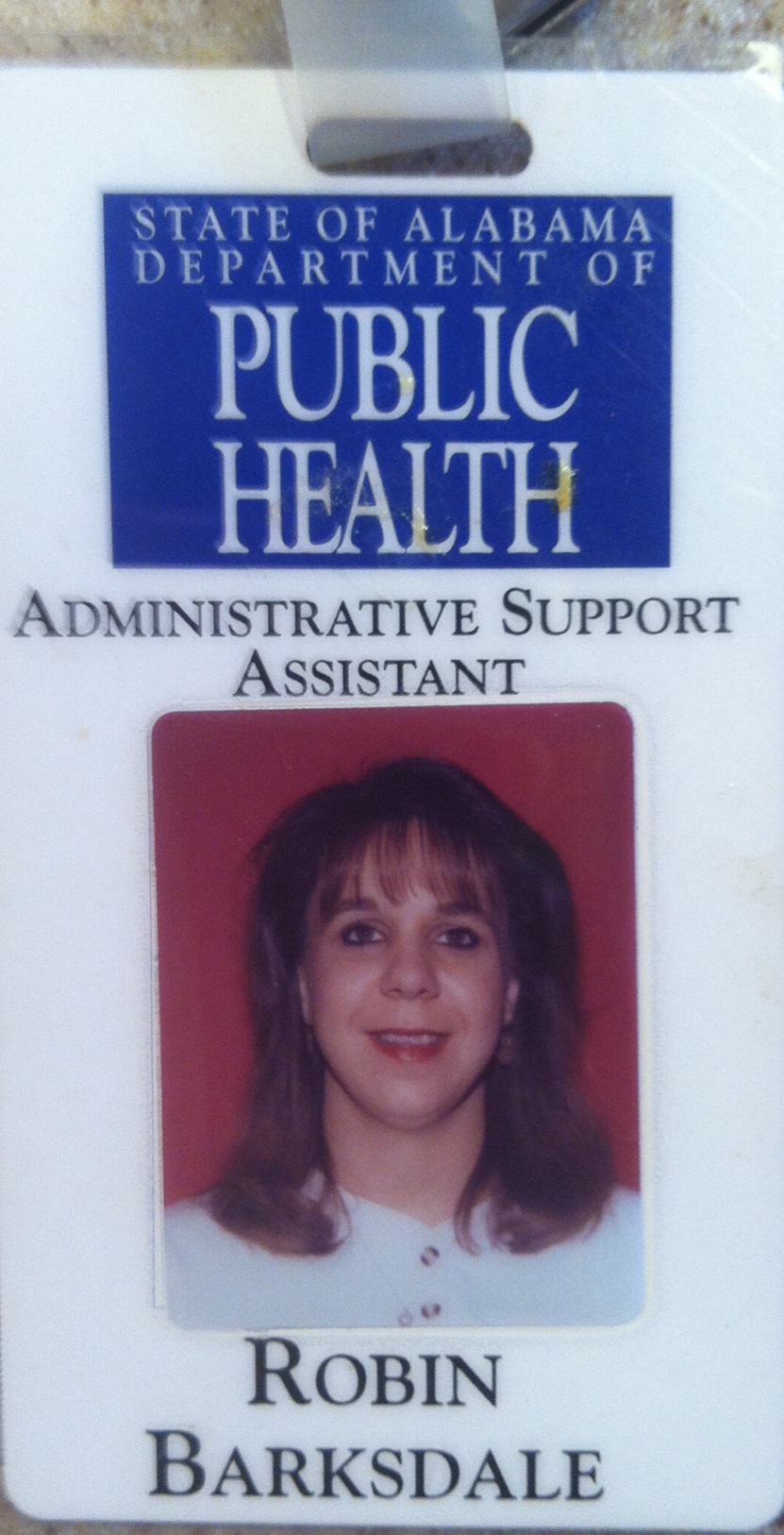In the center of the image is a full-color photograph of a white ID card for the State of Alabama Department of Public Health. The top portion of the ID card features a blue box with the white text "State of Alabama Department of Public Health." Below this, in black text, is the job title, "Administrative Support Assistant." The ID card includes a small, horizontally stretched, full-color photograph of a Caucasian woman with dark brown, shoulder-length hair and bangs reaching down to her eyebrows. She is wearing a white top and is positioned against a red background. At the bottom of the card, her name is printed in black text as "Robin Barksdale." The ID card has a hole at the top where a plastic loop allows it to be attached to a lanyard or clipped onto something. The photograph is positioned toward the center while the text elements are aligned in a vertical rectangle format. The overall setting is a clear and functional display of identification details.